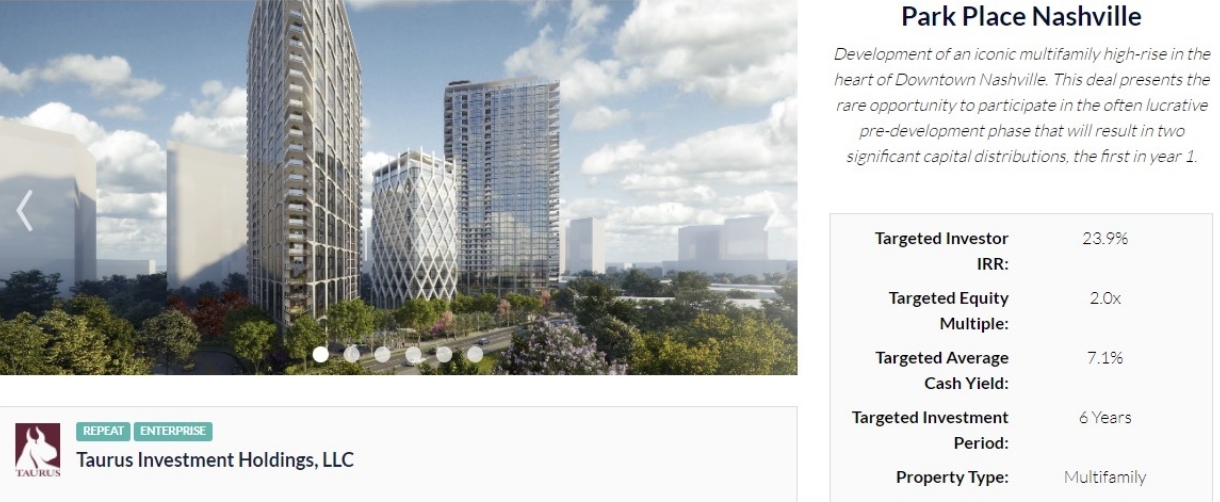A vibrant artist's rendering depicts futuristic office towers, part of an ambitious development project, set against a bright blue sky adorned with fluffy white clouds. The buildings are sheathed in reflective glass, mirroring the bustling vitality of their environment. At the base, a verdant canopy of trees adds an oasis-like charm, while the image is peppered with interactive dots likely offering various perspectives or close-up views on a web platform. The label below the image reveals the developer, Taurus Investment Holdings, LLC, marked by a sleek outline of a white bull set against a contrasting black and red background.

To the right, the text introduces "Park Place, Nashville," spotlighting the development of an iconic multifamily high-rise in downtown Nashville. This investment opportunity is uniquely poised for significant financial growth, with details specifying an anticipated Investor Internal Rate of Return (IRR) of 23.9%, a Targeted Equity Multiple of 2.0X, a Targeted Average Cash Yield of 7.1%, and a Targeted Investment Period of 6 years. The project is described as a multifamily property, illustrating a potentially lucrative entry into the pre-development phase with prospects for two substantial capital distributions within the first year.